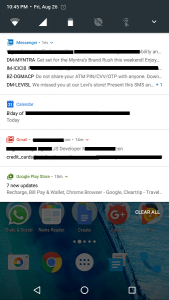This image is a detailed screenshot of a smartphone's notification panel taken at 10:45 p.m. on Friday, August 26th or 28th. The device is slightly below full battery and has a moderate Wi-Fi connection. The signal bars appear strong. There is an active alarm set.

Multiple notifications clutter the screen:
1. A message from DM Myntra promoting their Brand Rush event for the weekend, advising against sharing ATM PINs, and noting a missed visit to their Levi's store.
2. A calendar event for today, partially visible with details hidden.
3. An email from JB Developer in Gmail, also partially shown.
4. Notifications discussing sensitive details like credit card information, partially hidden.
5. Two updates from the Google Play Store mentioning recharge or billing for wallet services.

The dock at the bottom of the screenshot showcases frequently used apps such as WhatsApp, Chrome, Camera, and Google. The "Clear All" button, used for dismissing notifications, is also visible. The screenshot encapsulates the myriad of notifications and updates that can accumulate throughout a day, from messaging apps and calendar alerts to email updates and service notifications.